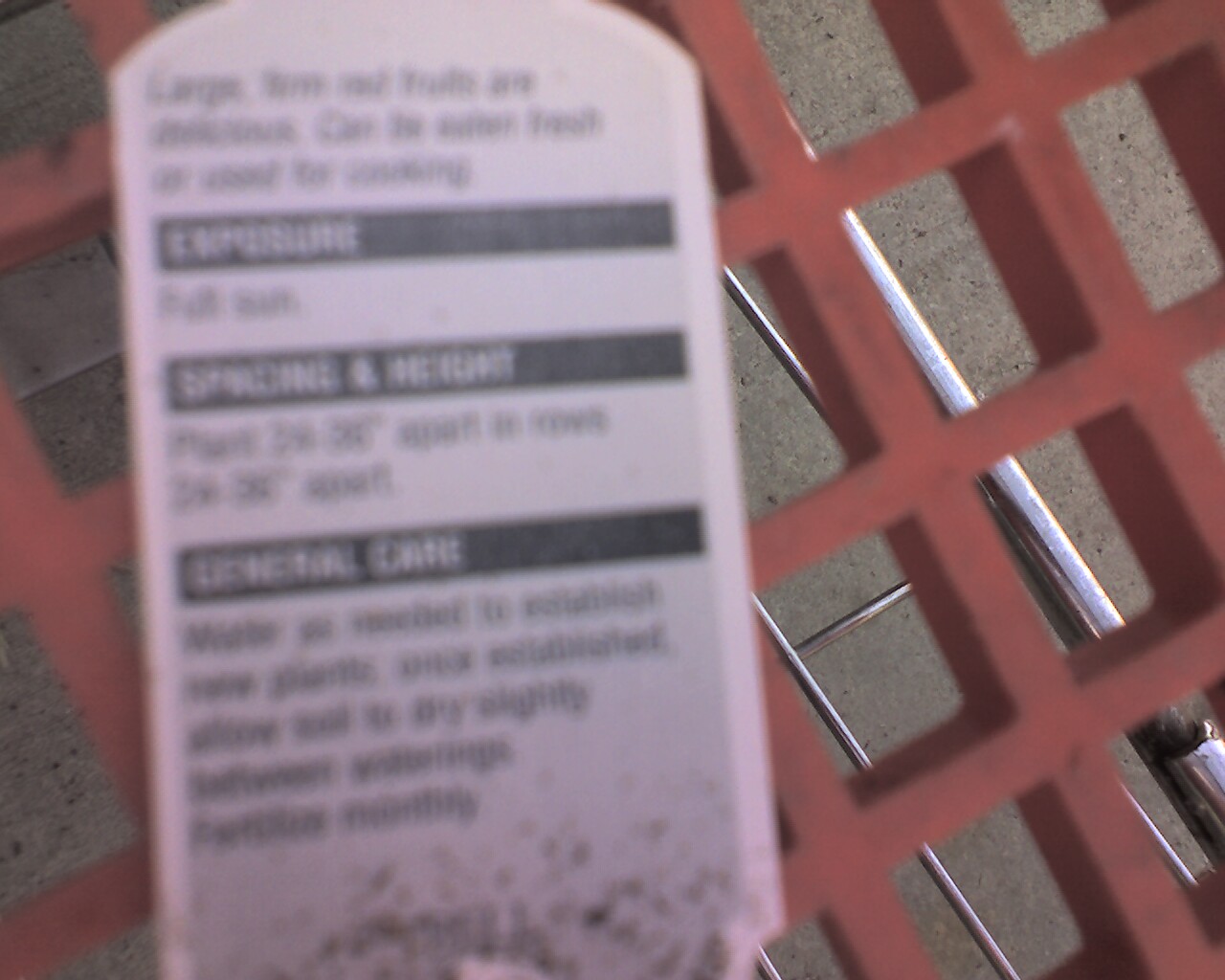This photograph captures a top-down view of a red plastic shopping cart, focusing on its intricate lattice pattern. Below the basket, the metal frame and lower shelf of the cart, typically used for bulky items like cartons of soft drinks, are visible. The cart is stationary on a silver concrete surface. A white tag, partially obscured by dirt and soil, lies atop the red plastic basket. Despite its blur, the tag appears to belong to a recently purchased plant and contains information on plant care, including exposure guidelines that recommend full sun. The tag also mentions height and general care instructions, providing a glimpse into the nature of the purchase.